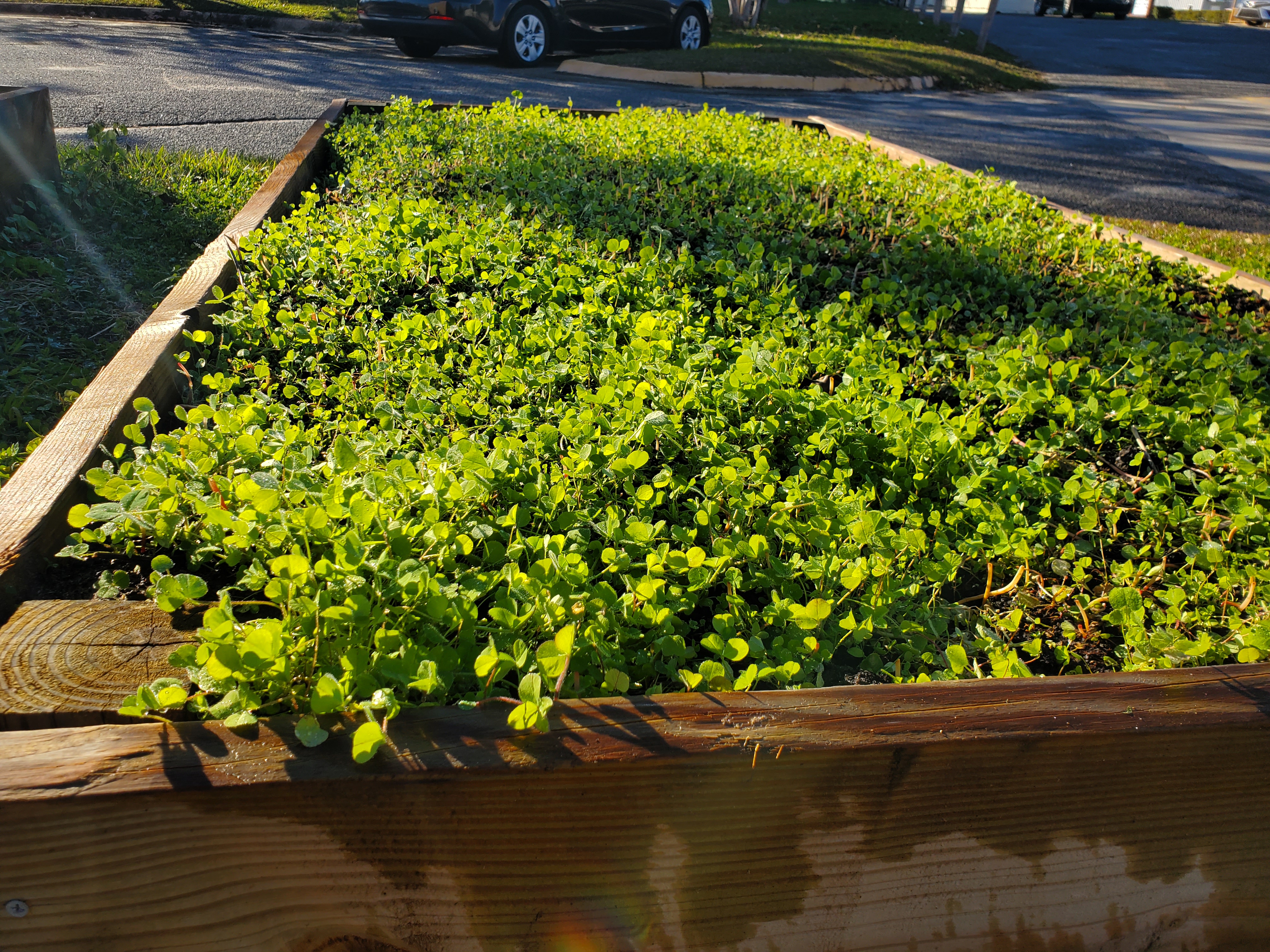The image depicts a large, elevated wooden planter box situated in a suburban yard. The box is filled with vibrant green shrubbery that can be inferred as an edible plant such as watercress, although specific identification is uncertain. The wooden frame of the planter shows signs of recent watering or rain, with water stains visible on its surface. Surrounding the planter is a neatly maintained grassy area, and just beyond this, a paved road is visible. A car is parked along the road, partially obscured by the shadows cast by nearby trees. The distant background features additional grassy knolls and a urban-suburban setting. Yellow-painted curbs enhance the street’s definition, contributing to the overall impression of a suburban allotment or garden space.